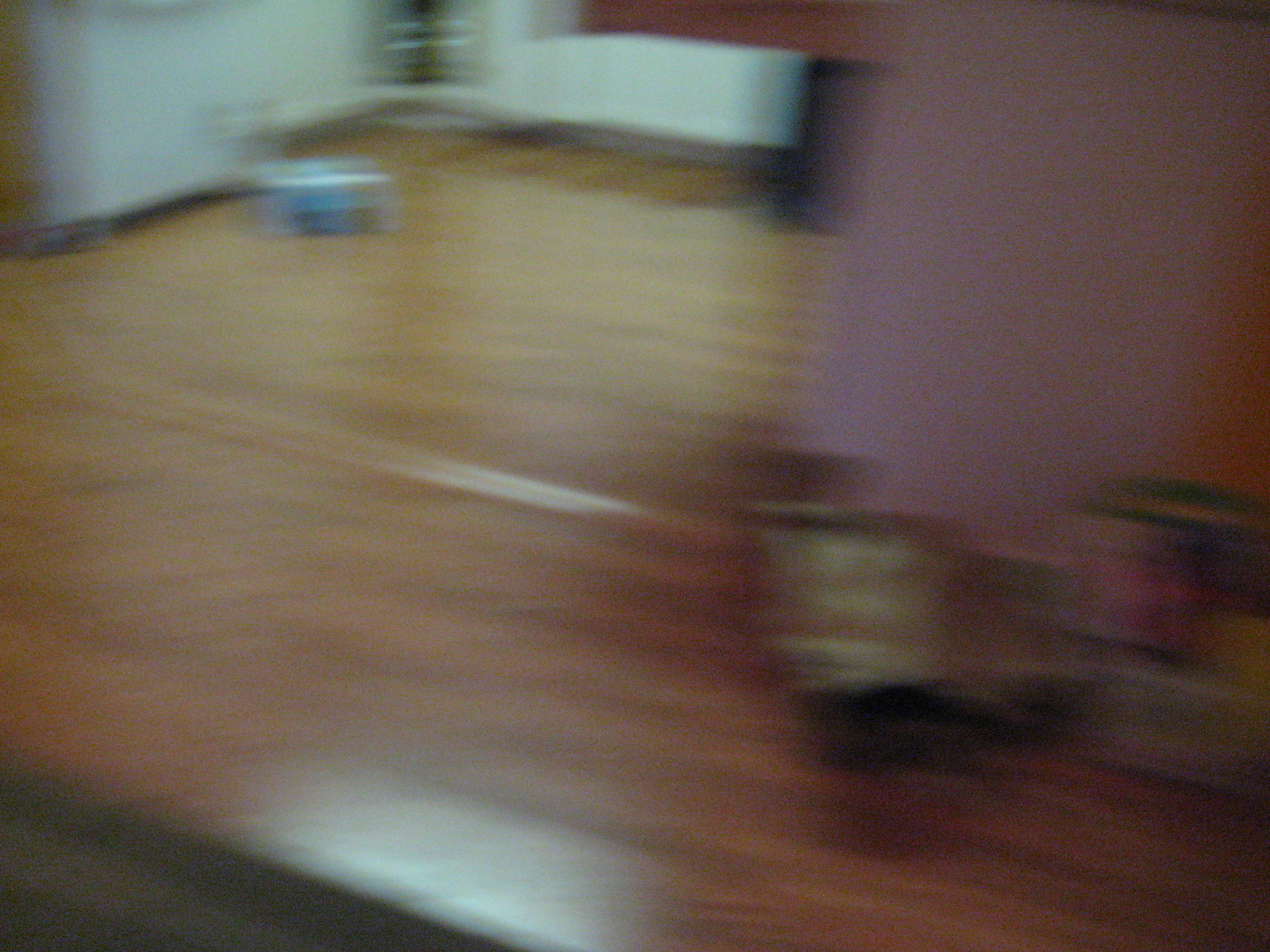This is a highly blurry color photograph, likely taken with a moving camera, making it challenging to decipher the exact details. In general, the background reveals what seems to be a hardwood floor extending to the back left or top left corner of the image. Towards the top left, there appears to be the bottom part of a white refrigerator, identifiable by a small hinge and a gap beneath it. In front of this refrigerator-like structure, there's a small, indistinct bluish and white blur which could either be a child’s blue plastic car or possibly a cat's water dish. 

Moving to the right side of the image, there's a vertical blur with a lavender hue, which might be part of a purple object or something else unclear due to the blurriness. Below this lavender blur, there's a rounded brownish shape that might be a person's pant leg and foot, suggesting someone might be walking to the right. Additionally, there's some ambiguity about a structure that could be a wall, cabinet, or even multiple items like cans or a dish towel hanging. In front of the lavender blur also appears to be what resembles large spools or cylinders in greenish and purple colors, though this detail remains vague due to the overall unclear nature of the image.